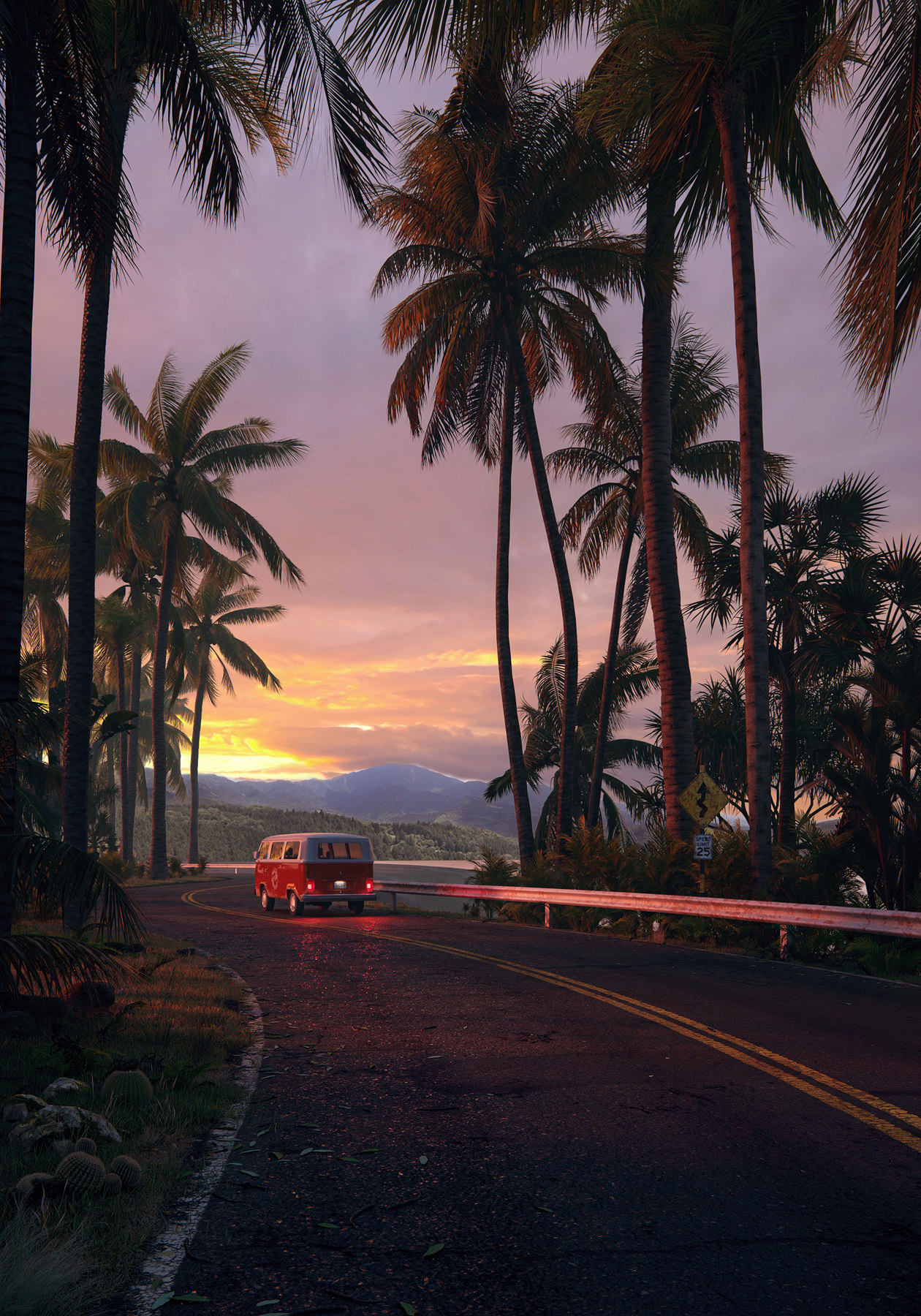The image depicts a nostalgic scene of an orange and white Volkswagen bus from the 1970s driving away on a winding two-lane road, flanked by tall palm trees. The road, which features a guardrail on the right side and a yellow road sign indicating curves ahead, leads toward a picturesque mountain range and green hills in the background, reminiscent of the Los Angeles Crest Mountains. The sky, bathed in the pastel hues of an enchanting sunset, transitions from yellow near the horizon to shades of orange, pink, and purple, with the sun barely setting behind the mountains. Small details like mushrooms by the roadside add to the charm. The headlights of the VW bus are turned on, capturing the moment just past dusk, creating an idyllic and postcard-perfect scene.